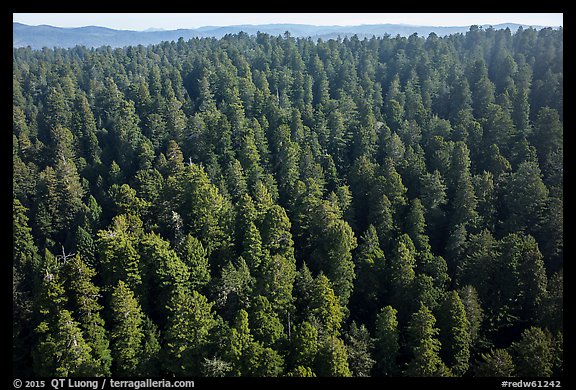This is an overhead aerial view of a dense forest captured by QT Luong in 2015, displayed on TerraGalleria.com. The image shows a sweeping expanse of over 100 green coniferous trees that cover 95% of the frame, blending into a distant, thin mountain ridge that extends from dark blue to light blue. Above the ridge, a small sliver of white sky is visible. The trees cast dark shadows, concealing any ground or structures below. The photograph includes a black border that reads "copyright 2015, QT Luong, TerraGalleria.com," and features a watermark, "#RedW61242," at the bottom.